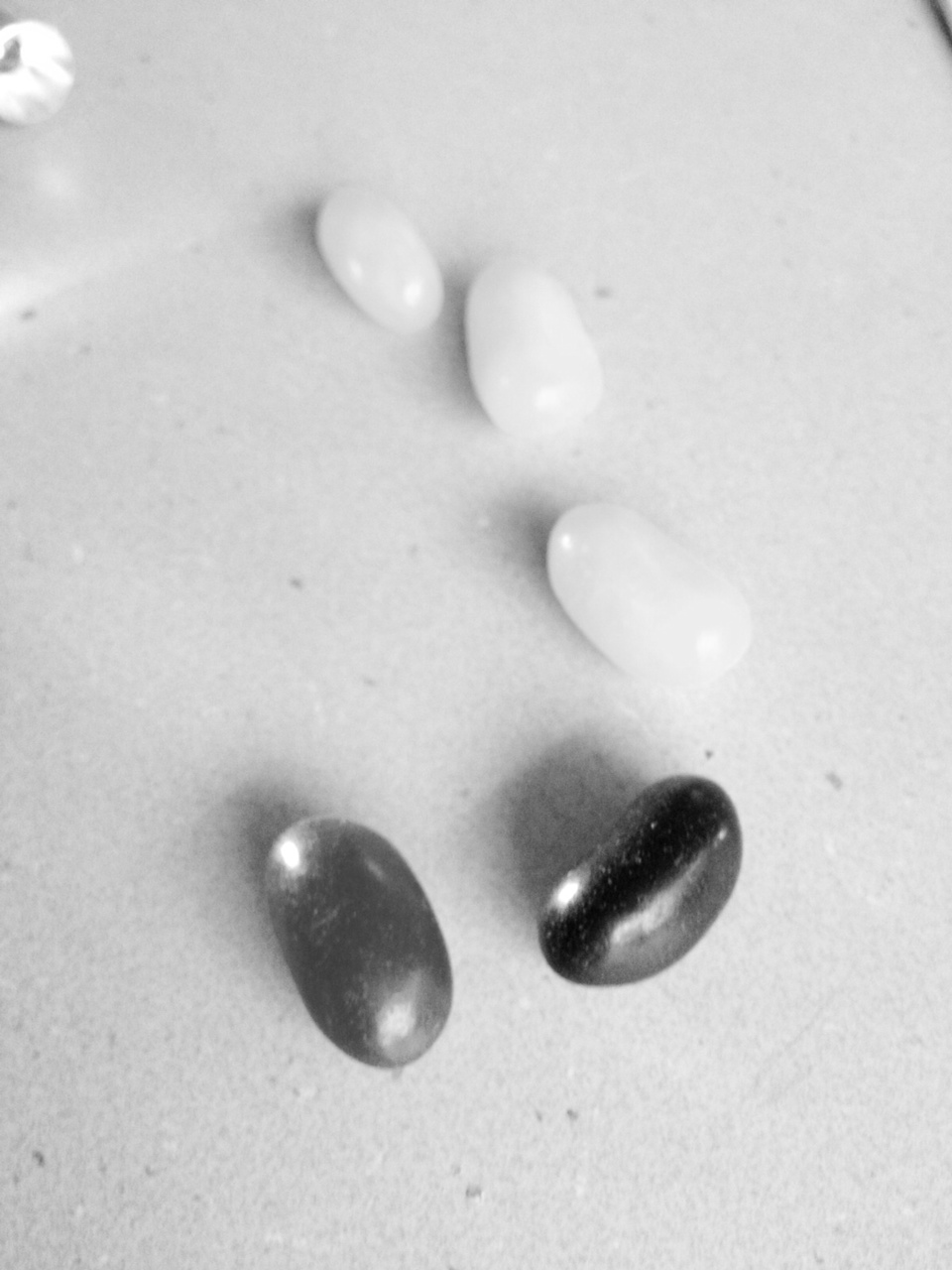This black and white photograph features a collection of five items resembling jellybeans, arranged diagonally from the top left to the center right, forming a curved line or reverse C shape. The scene is set against a solid white background, speckled with a few darker gray spots, as if something had dripped onto it. The image is taken from a top view, showcasing the distinct appearances of these objects: three polished, white stones that are oval-like and shiny, and two darker, kidney bean-shaped stones that resemble river rocks. The darker stones, with shades ranging from dark gray to charcoal gray, are placed beneath the lighter ones. In the upper left corner, there’s a small, circular object with a fluted edge resembling a bottle cap from a glass bottle. Overall, the arrangement of the stones seems random, adding a touch of natural disorder to the composition.